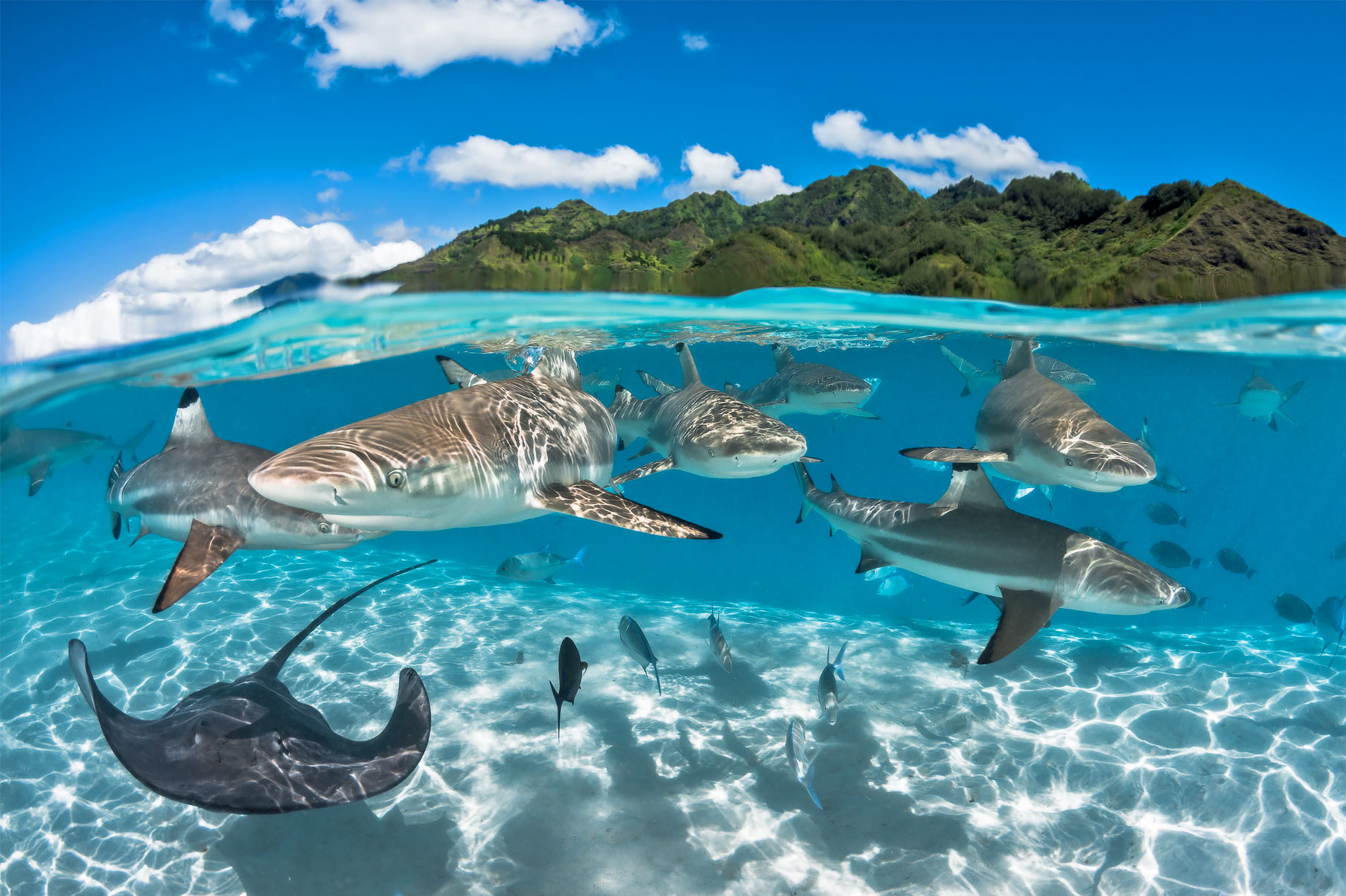This is a stunning landscape photograph featuring an island and the waters surrounding it, cleverly capturing both above and below the waterline. Above the water, there is a picturesque island on the left, blanketed in verdant greenery. The backdrop showcases a brilliant blue sky dotted with a few prominent white clouds. Below the water's crystal-clear surface, a captivating underwater scene unfolds with a pristine, sandy base illuminated by sunlight. Various sea creatures glide through the water, including six different sharks, such as hammerheads, accompanied by a stingray in the bottom right and a school of fish. The vibrant marine life and clarity of the water create an aquarium-like appearance, lending an almost surreal quality to the image. The juxtaposition of the serene, natural landscape above with the lively activity below contributes to the photo's mesmerizing and somewhat uncanny allure, rendered with such precision it almost appears AI-generated.